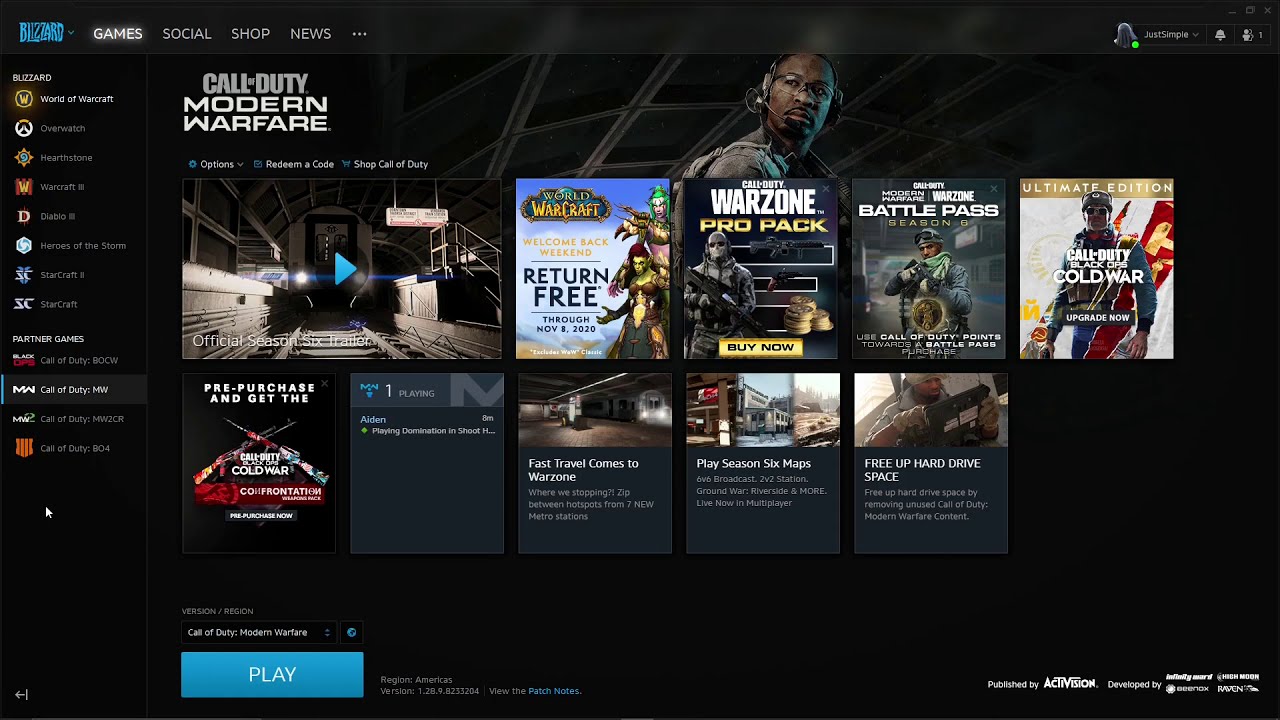The image features a user interface with a black background. At the top, there is a navigation bar with a small blue box labeled "Games," which is highlighted, alongside other categories such as "Social," "Shop," and "News," followed by three dots indicating more options. On the right side of the top bar, there's a small blue dot with a white icon inside it.

To the left, there's a vertical list, each line accompanied by small icons. At the bottom of the list, an upwards-pointing arrow is visible. On the right side of the image, the title "Call of Duty: Modern Warfare" is displayed in white text next to a small blue dot.

In the central portion of the image, a large room is depicted, marked by a blue arrow pointing to the right. The words "pre-purchase" are visible, along with a reference to "Cold War" and an image of a red vehicle. Below this, a gray box with blue accents displays a "1" and an "M."

At the top again, the title "Warcraft" is shown with the phrase "return free." Below, "Warzone Pro Pack" with a "buy now" option is displayed. Further details include "Battle Pass" and "Call of Duty: Cold War - the Ultimate Edition." At the bottom, the text "Play Season 6 maps and free hard drive space" is visible next to a blue play button, with additional white text beneath it.